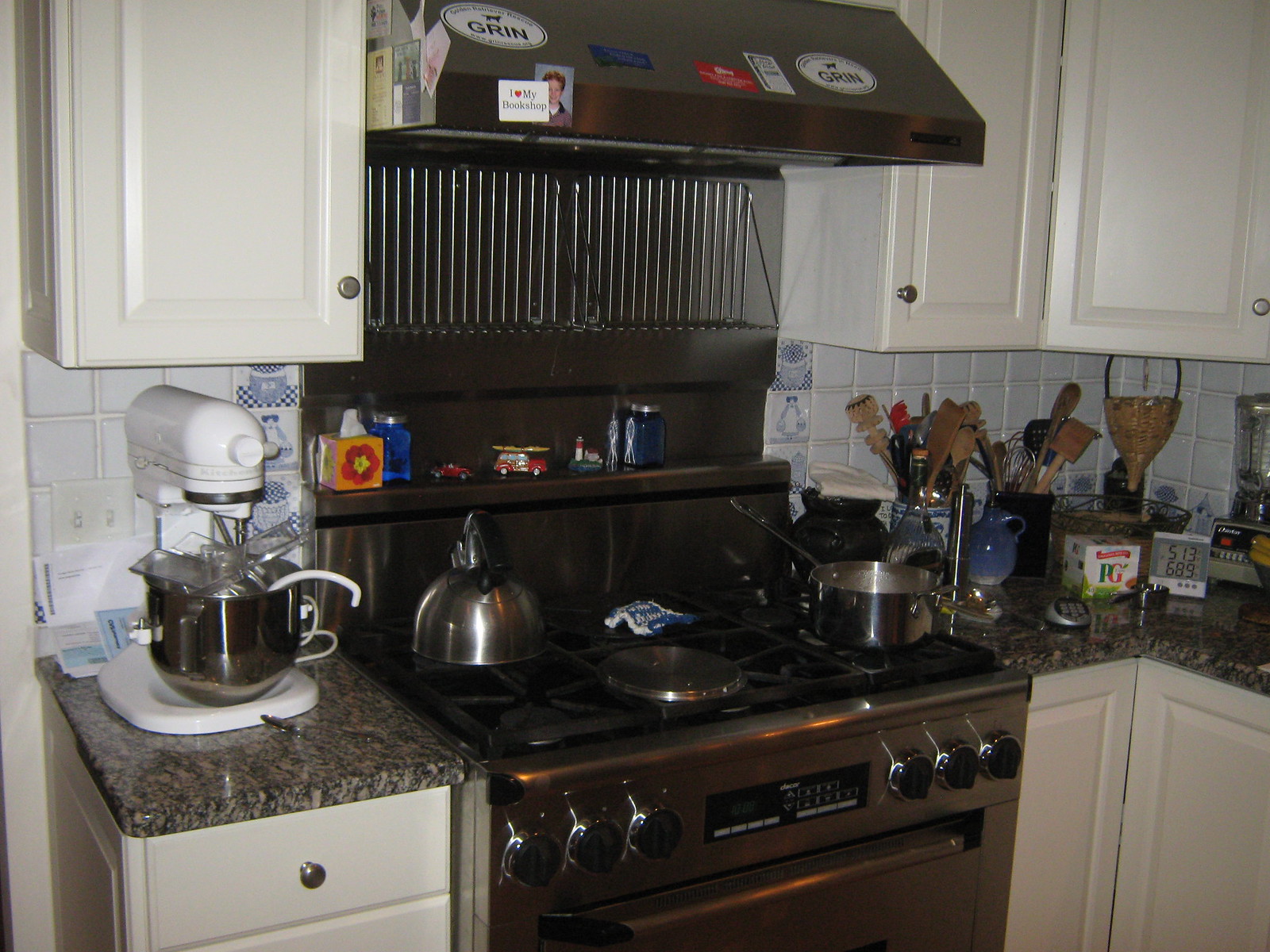This image depicts a modern kitchen interior, characterized by sleek white cabinetry and a speckled gray and black stainless steel countertop. On the left side of the image, a white stand mixer is positioned beneath the upper cabinets, which might initially be confused with a coffee machine due to its design. Moving right, a stainless steel stove with four burners is the focal point, accompanied by various pots, pans, and a kettle on top. Adjacent to the stove is a collection of kitchen utensils, including spatulas, organized for easy access. Both above and below, white cabinets provide ample storage space. A stainless steel oven hood occupies the space above the stove, while various small kitchen products are sporadically placed, reinforcing the image as a functional and well-utilized kitchen space.